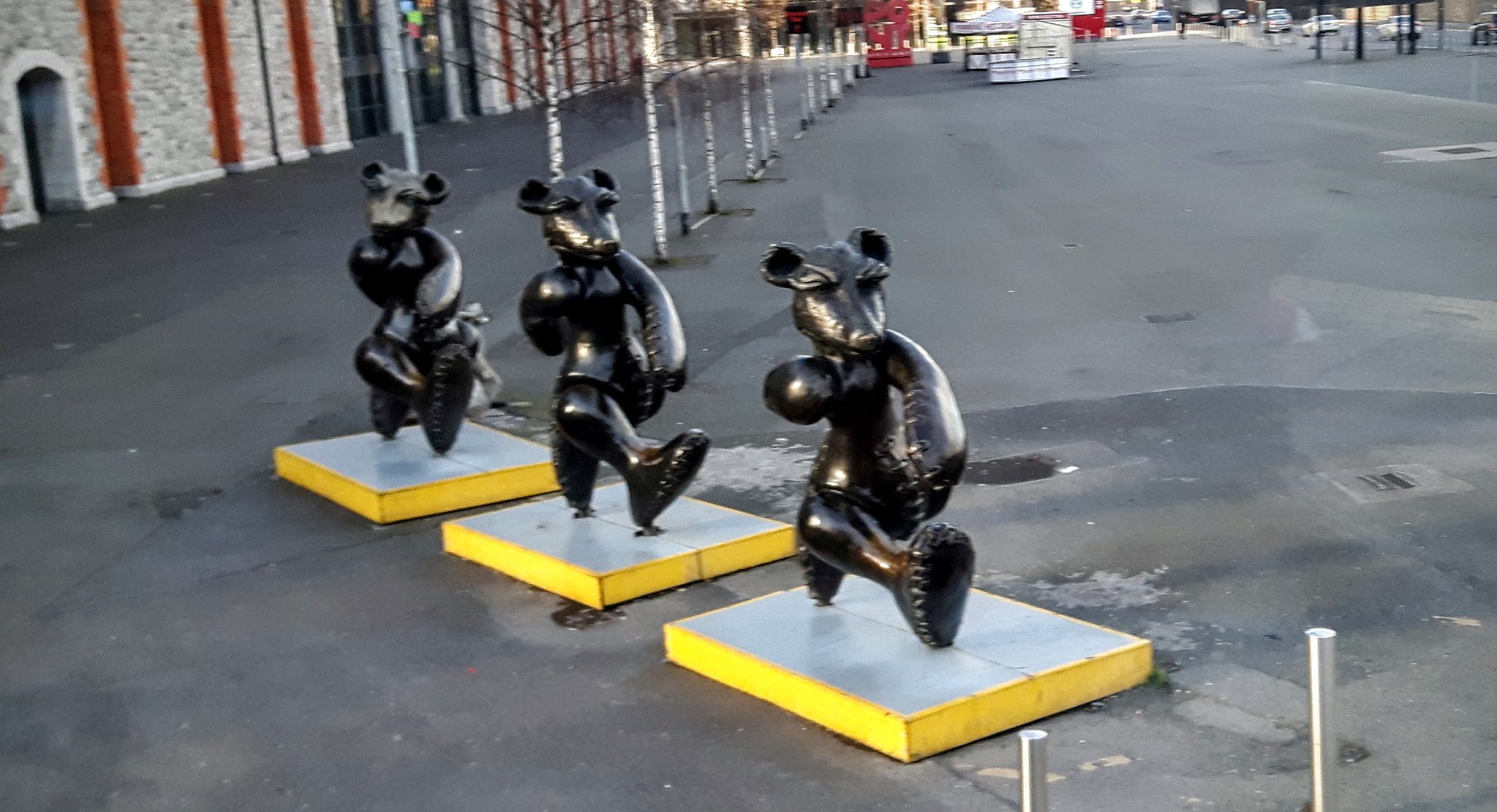The image is a color photograph in a landscape orientation, featuring an outdoor public display of three anthropomorphized bear statues. Set against a large, tarmac-covered square or gathering area, the statues are positioned on rectangular platforms. These platforms, aligned diagonally from the bottom right to the back left, have yellow edges and silver-grey tops. The black statues, possibly made of metal or dark bronze, depict bears in motion with their feet tipped upward as if walking. Each bear has a rounded, pronounced front, giving an impression of bloated chests, and features stubby, ball-like arms. Their heads are turned in different directions: the bear at the back looks to the right, the middle one gazes forward, and the front bear appears to look downward.

To the left, a row of very thin, white-barked trees extends into the distance, separating the artworks from a sidewalk bordered by a large stone building with archways. The background features additional structures and hints of market stalls, along with some traffic. The ground has a dark grey color with a mix of smooth and rough patches. Near the bottom right corner of the image, metal poles protrude from the ground. The scene is reminiscent of a town square with a somewhat eclectic mix of elements, including castle-like architecture and urban fixtures, creating an intriguing, almost surreal juxtaposition.